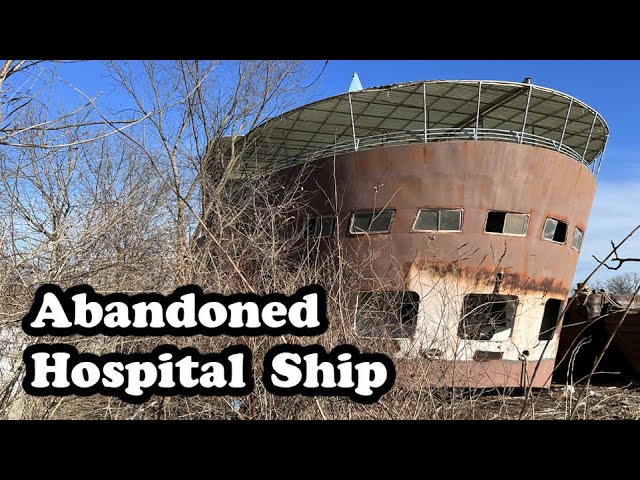This color photograph, in landscape orientation, depicts an abandoned hospital ship run aground in an open field, surrounded by dead trees and shrubbery, suggesting wintertime. Dominating the right side of the image, the large elliptical ship exhibits a rusty, reddish-brown hue, with a lighter patch of white around the bottom three windows, transitioning into rust as it ascends. The front of the ship features numerous windows and an arched railing balcony with a covering on top. A light blue triangle is visible at the ship's apex. The stark blue sky contrasts with the ship's deteriorating structure. Bold white text, outlined in black, across the bottom left of the image reads "Abandoned Hospital Ship," overlaid on the sparse, lifeless vegetation. The photograph utilizes representational realism with integrated typography to emphasize the haunting abandonment of this once-functional vessel.